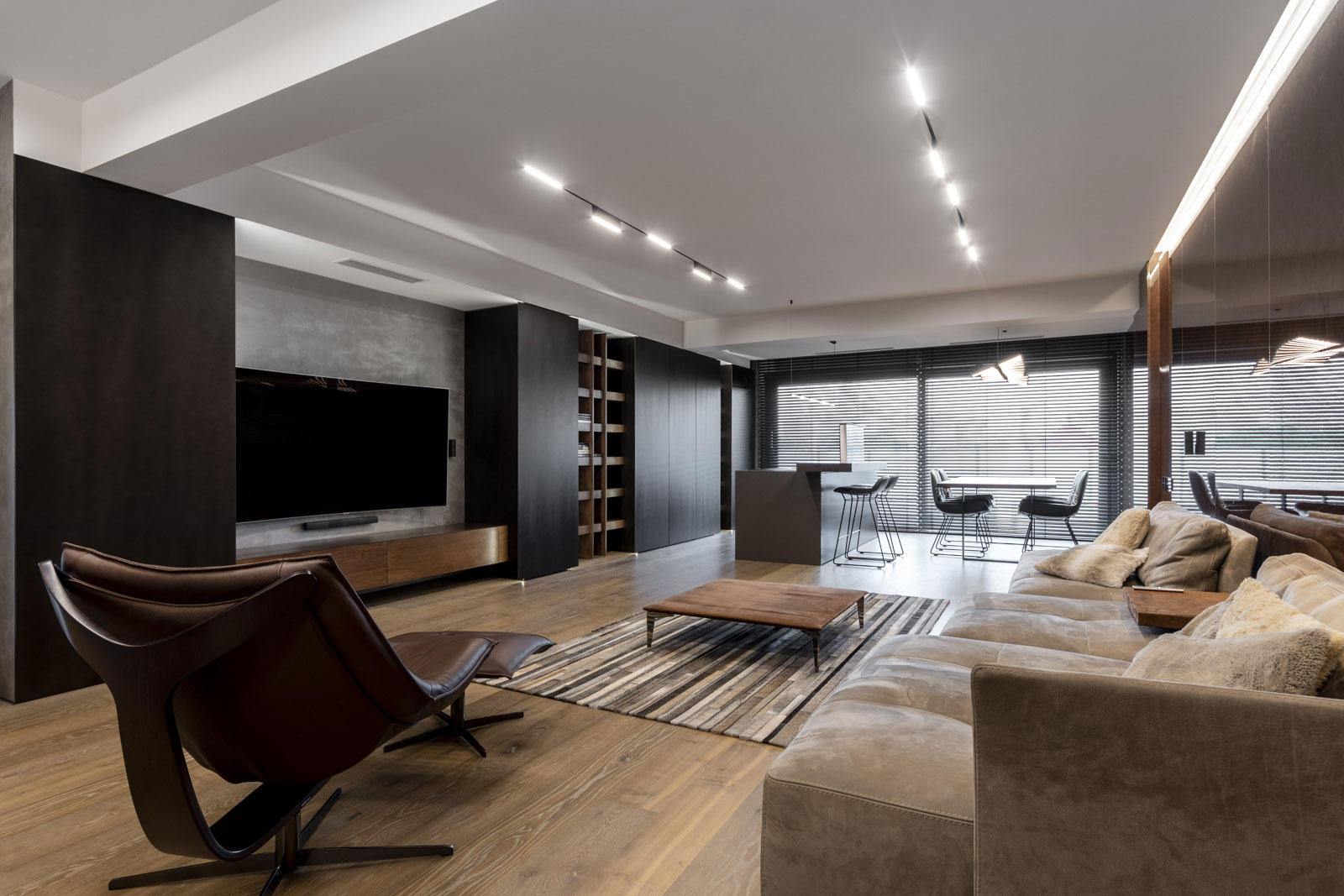This is an image of a modern, stylish living room that could also function as an office break room. The room features wooden floors and a soft beige couch with fluffy, cotton-like pillows on the right side. Across from the couch is a unique, futuristic leather recliner, characterized by its flat, geometric design and metal supports. To the left, a large flat-screen TV is mounted on a gray concrete wall above a wooden cabinet, flanked by sleek, handle-less floor-to-ceiling storage cabinets painted black. A low ceiling with thin recessed lights adds to the room's cozy ambiance.

In the background, you can see a bar area equipped with a small countertop and barstools, which transitions to a dining area featuring a rectangular table with four grey chairs. Large windows with thin black frames allow natural light to filter through. The overall décor employs neutral beige and brown tones, creating a harmonious and modern aesthetic in this well-designed space.